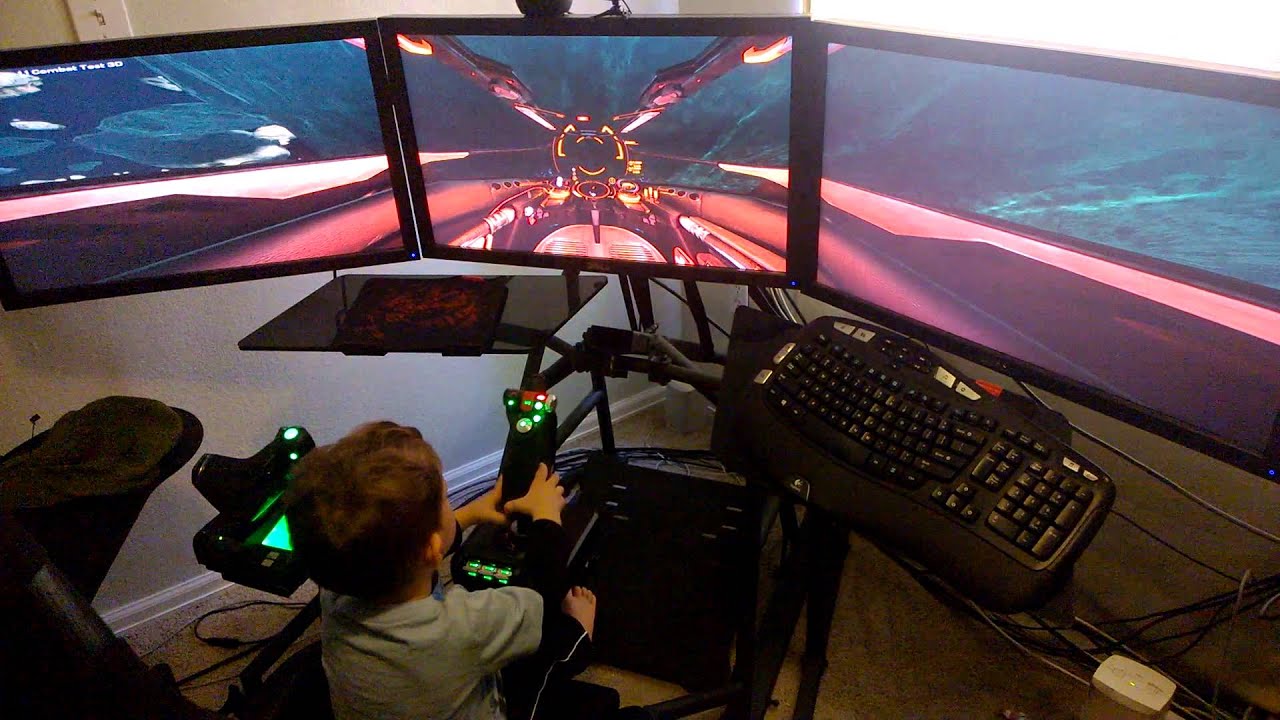In the image, a young boy with short brown hair is immersed in an elaborate gaming setup in his bedroom. He is seated in a high-tech gaming chair, focused intently on a triple-monitor display that spans the top portion of the frame, showing a video game featuring a spaceship in outer space. The screens have no text and display vivid colors including blue, dark blue, pink, turquoise, and green. 

The boy is using a sophisticated controller, a black joystick with green and red lights, which is positioned centrally in front of him. Nearby, to the right, there is a black keyboard and a mouse pad set on a glass table. An illuminated green keypad is visible on the left side. The room has white walls, a light switch in the top left corner, and a tan rug on the floor. The boy, casually dressed in a t-shirt and pants, seems very engaged in his gaming experience, surrounded by the array of equipment.